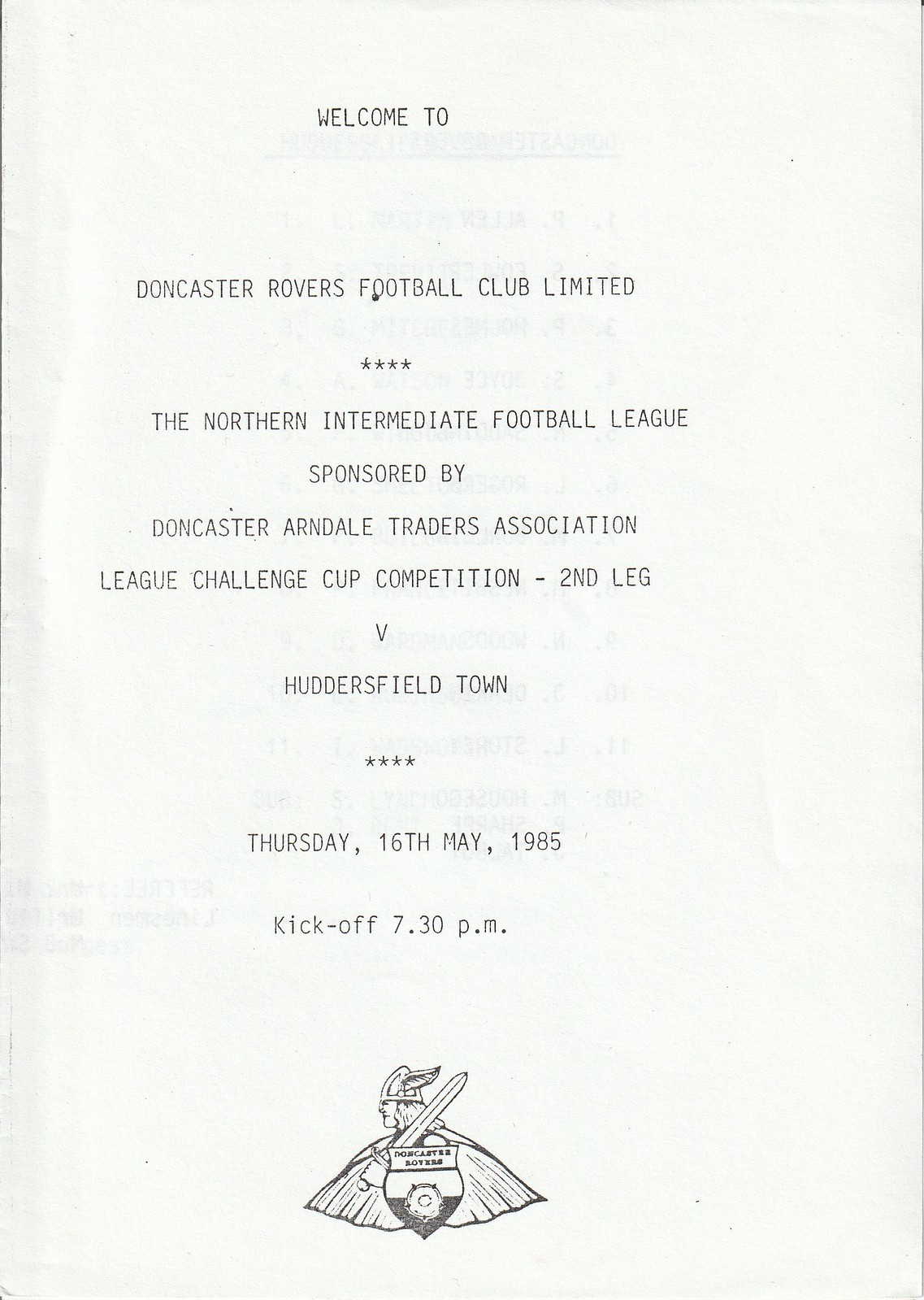This black-and-white welcome pamphlet invites attendees to a UK football game between Doncaster Rovers Football Club and Huddersfield Town. It is part of the Northern Intermediate Football League Challenge Cup Competition, Second Leg, sponsored by the Doncaster Arundel Traders Association. The event is scheduled for Thursday, 16th May 1985, with kickoff at 7:30 PM. The pamphlet features the Doncaster Rovers logo prominently at the bottom, depicting a man in a Viking helmet, wielding a sword and donning a large cape, possibly with wings encircling a shield. The white background hints at its thin paper material, allowing some text from the next page to be visible.